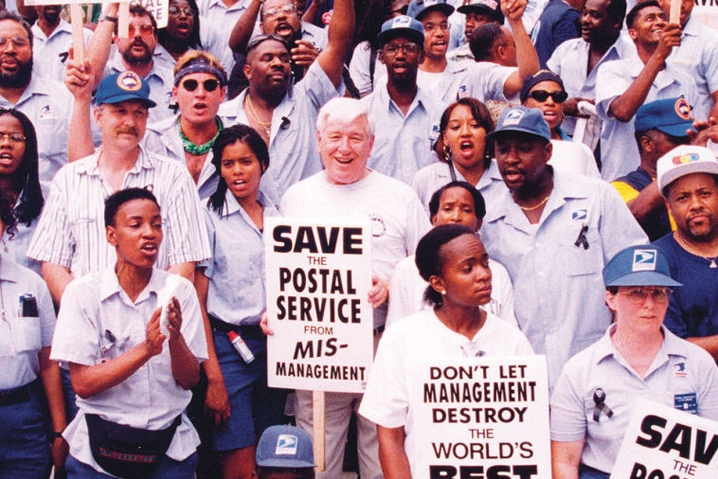The picture, taken a couple of decades ago, captures a large, peaceful demonstration of postal service workers and supporters, all clad in their uniforms, including postal caps and white shirts. They are gathered in unity to protest against mismanagement within the Postal Service. Many participants are seen holding signs aloft, some with fists raised in solidarity. Prominent among the signs are messages like "Save the Postal Service from Mismanagement" and "Don't let management destroy the world's best." The gathering is marked by a mix of expressions, from unhappy to determined, with both men and women, including a notable white-haired man and a young Black woman, clearly visible among the crowd. The atmosphere is one of collective resolve, as the participants cheer, clap, and raise their signs high, embodying their commitment to preserving the integrity of the Postal Service.